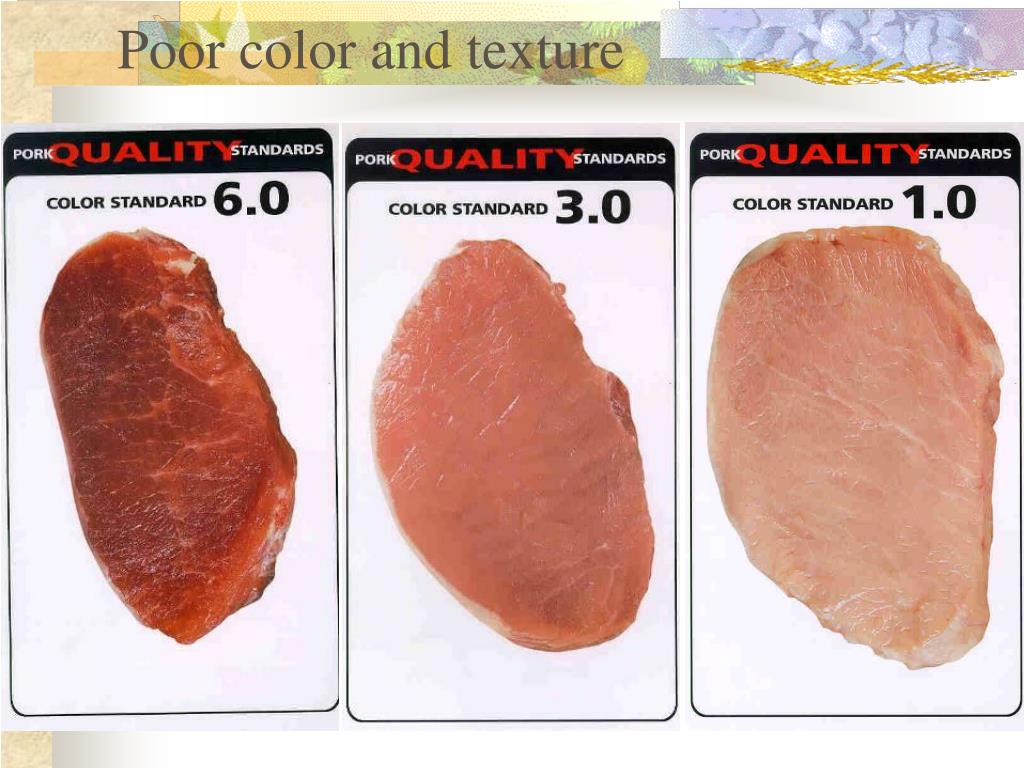This image appears to be a slide from a presentation demonstrating pork quality standards through color comparison. At the top of the slide, in black text, is the title "Poor Color and Texture." Below this header, the slide features three rectangular paper trays, each holding a piece of boneless pork with minimal fat. Above the trays, in a multicolor textured background, is the label "Pork Quality Standards," with the word "pork" in white, "quality" in red, and "standards" in white text. 

From left to right, the trays showcase pork with varying color standards:
- The left tray holds a darker, reddish-pink piece of pork labeled "Color Standard 6.0" in black text.
- The middle tray contains a lighter pink pork piece labeled "Color Standard 3.0" in the same black text format.
- The right tray features a very light pink, almost white, pork piece labeled "Color Standard 1.0" in black text.

This detailed and organized visual clearly communicates the gradation in pork color standards.